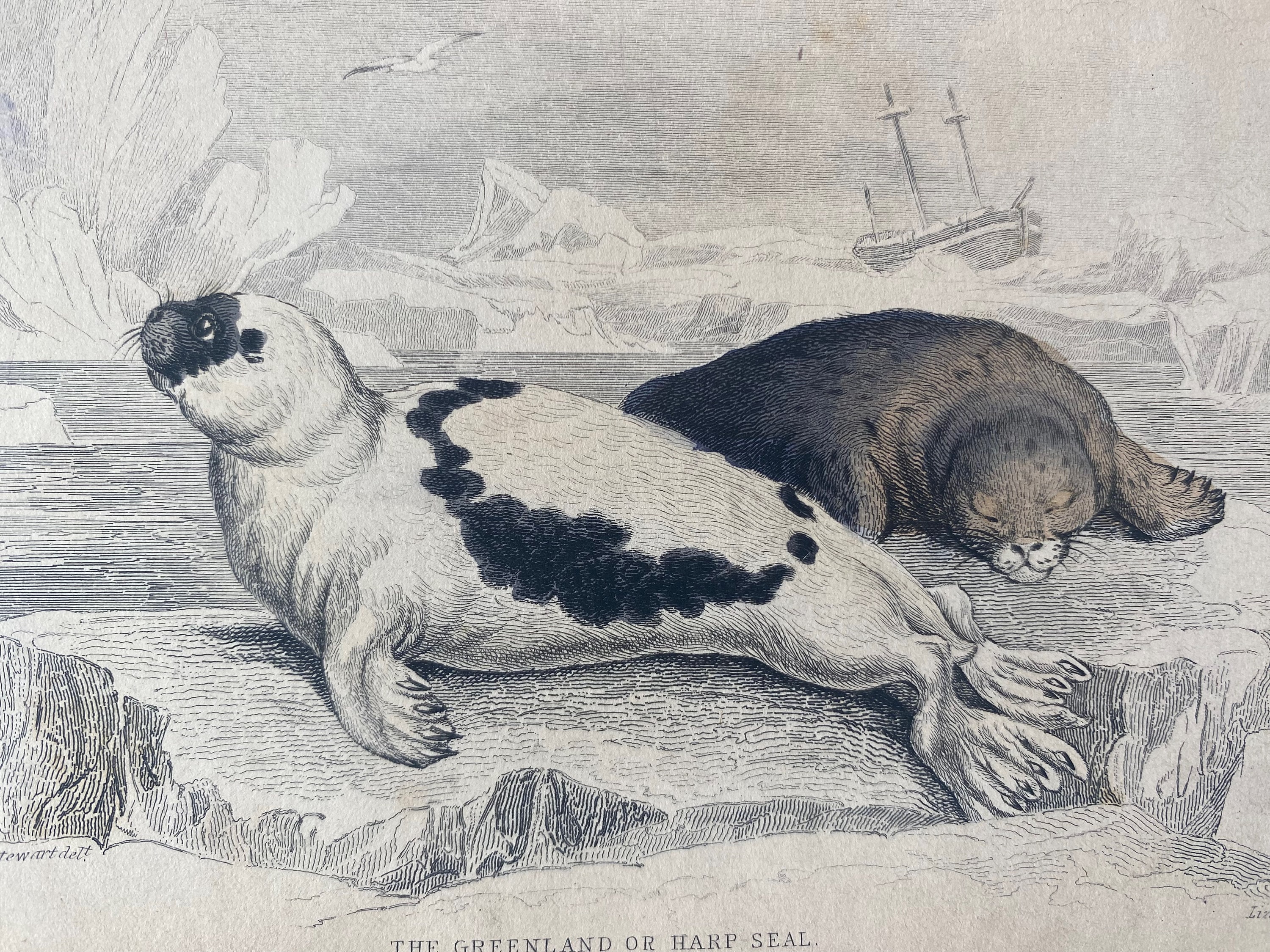The vintage-style drawing, primarily in black and white with hints of brown texture, depicts a serene Arctic scene. In the foreground, on a detailed iceberg, rest two seals – one a white seal with black spots, looking up at the sky, and the other a darker brownish-gray seal, seemingly asleep. The surrounding icy landscape features peaks of ice and an icy ocean stretching into the horizon. Flying seagulls dot the sky, adding to the sense of wilderness. In the background, a ship with two sails and three crosses on its body appears stranded amidst the icebergs, stuck in the frozen sea. The text at the bottom of the image reads, "The Greenland or Harp Seal," indicating the species of the portrayed seals. This intricate artwork captures the stark beauty of the seals' natural habitat.